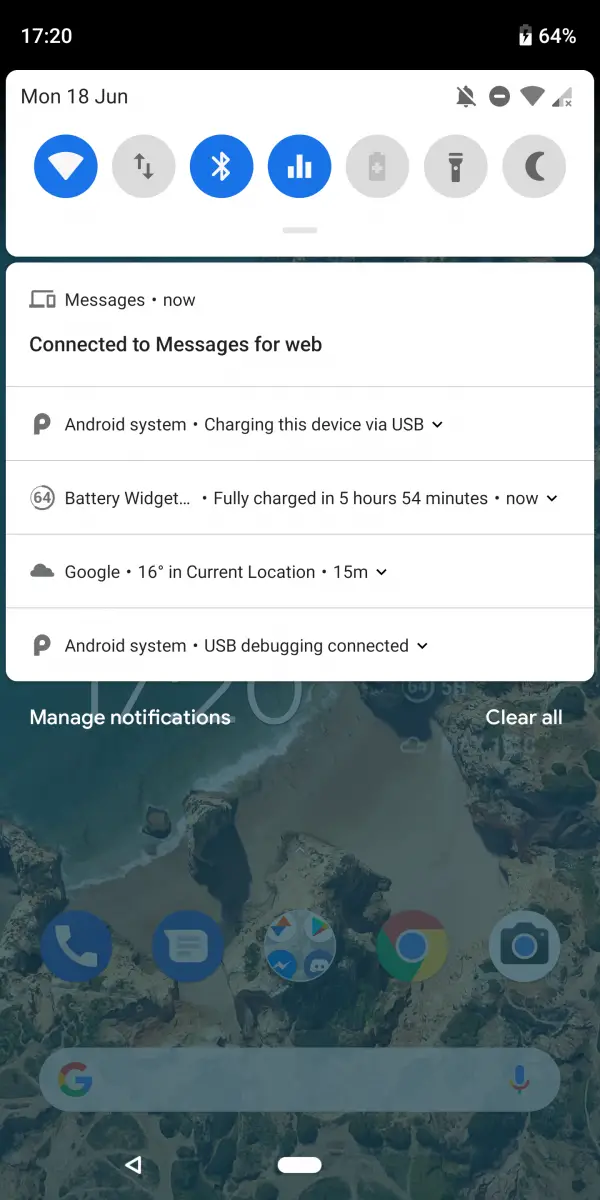A screen capture of a smartphone displaying the quick settings and notifications menu. The screen shows the typical quick access buttons for toggling Wi-Fi, cellular data, Bluetooth, flashlight, battery saver, and dark mode. At the top of the screen, the time is displayed as 17:20 and the battery indicator shows 64% remaining. 

The background of the phone is dimmed as the user has pulled down the menu from the top. The status shows that Do Not Disturb mode is activated and notifications are turned off. The phone is connected to a Wi-Fi network but has no cellular service, likely due to the Wi-Fi connection.

Several notifications are visible, indicating various statuses and updates:
- Messages are connected to Messages for Web.
- An Android system notification stating the device is charging via USB and will be fully charged in 5 hours and 54 minutes.
- A Google notification indicating the current temperature at the user’s location is 16 degrees Celsius, recorded 15 minutes ago.
- Another Android system notification indicating USB debugging is connected.

At the bottom of the menu, there are options to 'Manage notifications' and 'Clear all'. The notification bar occupies approximately the top half of the screen, with the dimmed background of the phone visible underneath.